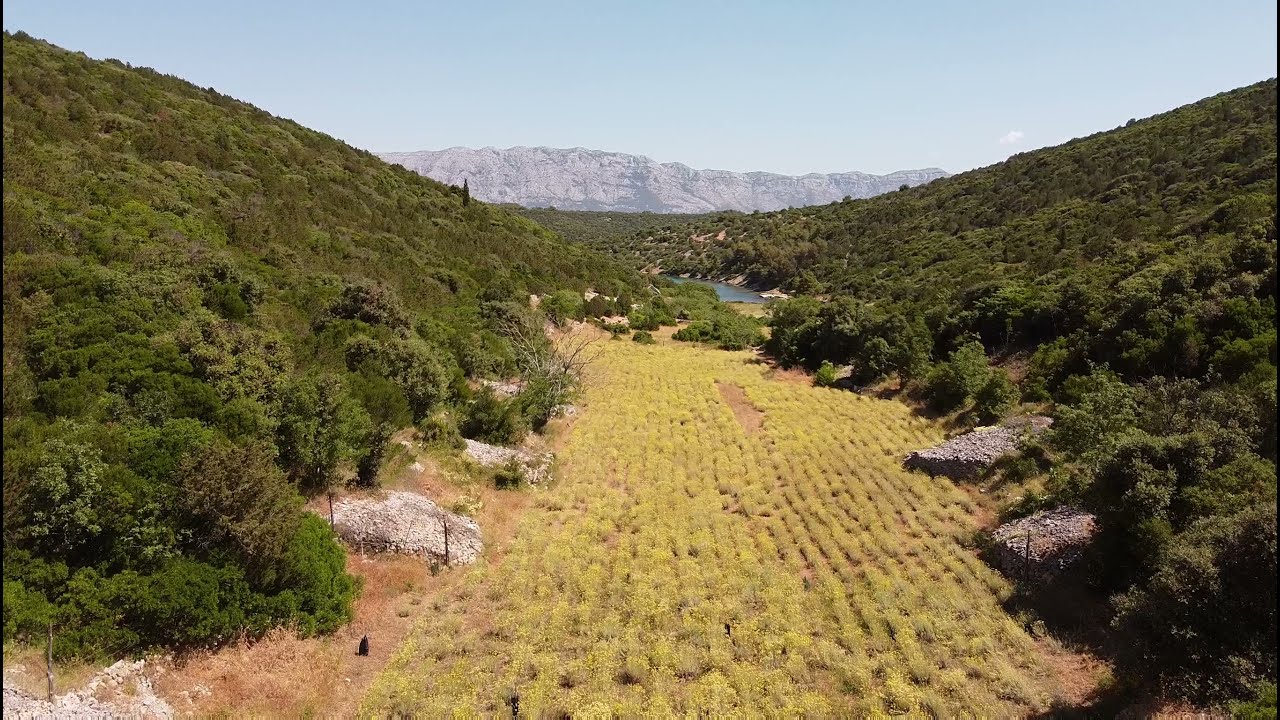This daytime outdoor digital photograph captures an elevated view of a serene valley bordered by low, green, bushy tree-covered hills on both sides. In the center of the valley, neat rows of light yellow flowering bushes stretch towards a small blue waterway, possibly a pond or river, which reflects the vibrant surroundings. Light-colored gravel piles are sporadically placed at the base of the hills, adding texture to the scene. In the background, where the hills converge, a rocky mountaintop rises majestically, framed by a clear, bright blue sky without a hint of clouds. The overall composition, viewed likely from a drone, highlights the peacefulness and natural beauty of the landscape, with its intentional rows of yellow shrubs leading the eye towards the distant mountains.